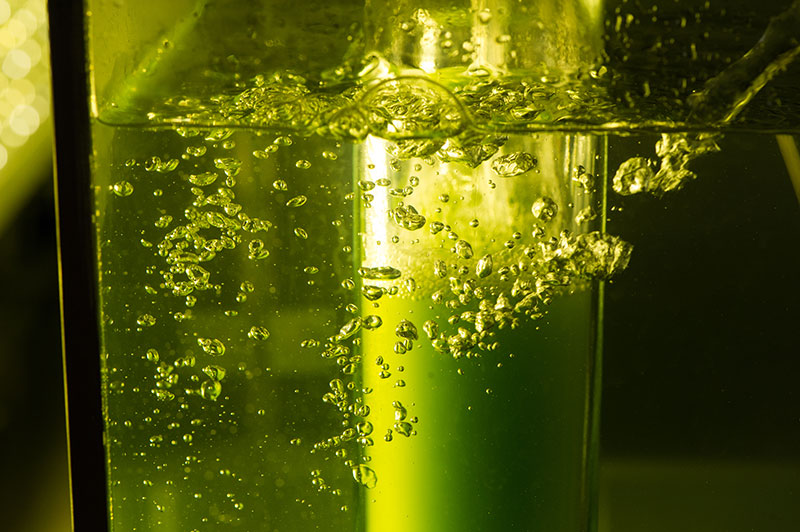This is an up-close photo of a clear liquid inside a glass container, appearing as if it's tinted with a dark, almost neon green color. The liquid is visibly bubbling with numerous small bubbles rising to the surface, creating a dynamic, effervescent effect throughout the image. The container, which seems to resemble either a regular drinking glass or a fish tank, has a distinct, dark edge that frames the scene. Within the glass, a central tube-like object, reminiscent of a filtration device commonly found in aquariums, is partially submerged, contributing to the effervescent activity. The entire image has a translucent quality, with all elements, including the liquid, container, and central object, bathed in a consistent green hue. The top right of the photo reveals the surface of the water and a small stream of water pouring into the container, enhancing the sense of continuous motion and interaction within this green-tinted aqueous environment.